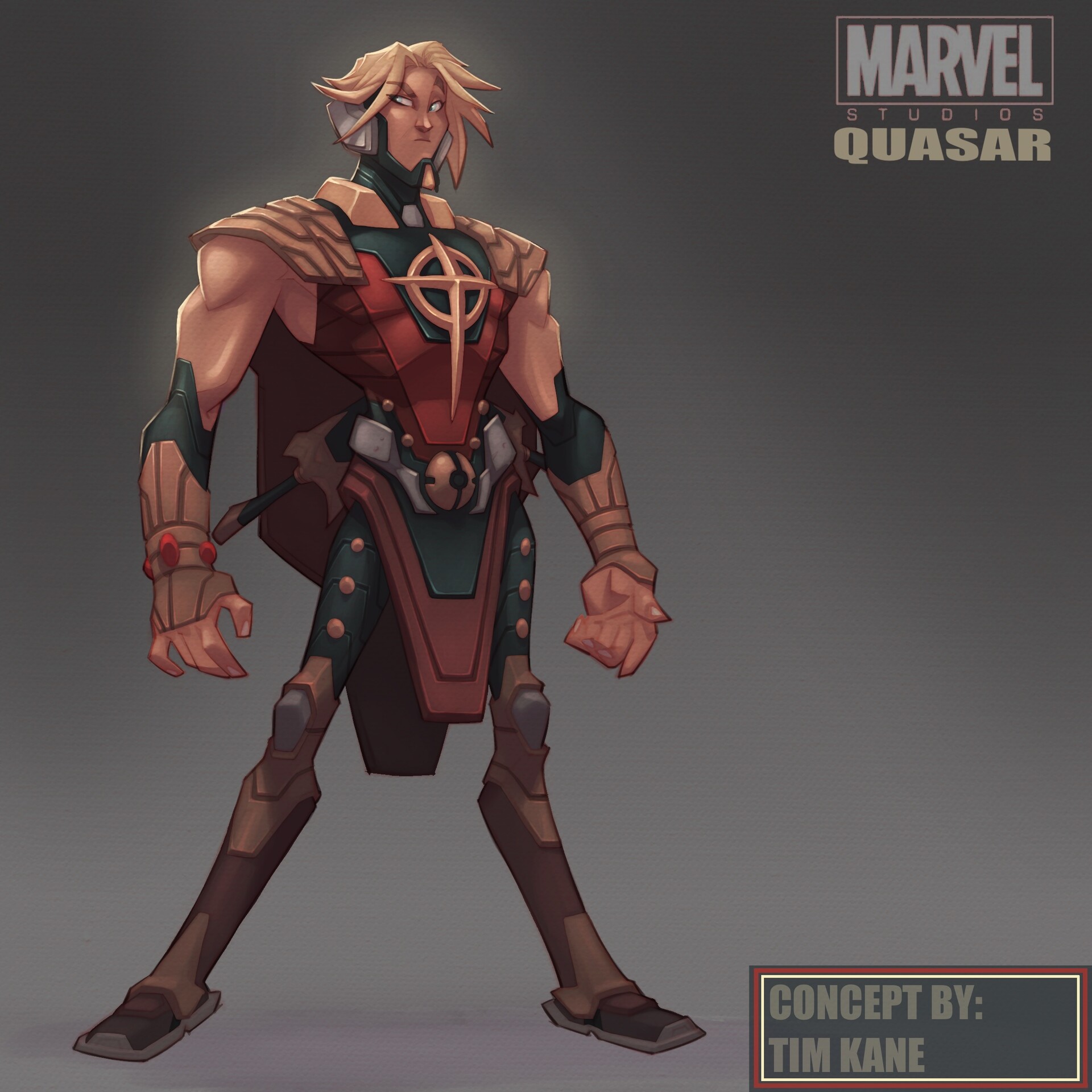The image showcases concept art for a Marvel Studios character named Quasar, created by Tim Kaine. The background is a plain gray, highlighting the central figure. In the upper right corner, the iconic Marvel logo is displayed in gray letters, with "Studios" and "Quasar" written below. The bottom right corner features a darker gray box trimmed with narrow tan and wider red bands, and an outer black band. Inside the box, the text reads "Concept by Tim Kaine."

The character stands with an imposing presence, featuring mid-length, spiky blonde hair extending to the chin. The figure is clad in a futuristic suit of armor with a medieval flair, predominantly in shades of copper, maroon, and red. A stylized copper cross set against a dark green background is prominently displayed on the chest, resembling the NATO symbol. Additional details include brown thigh-high boots, green pants adorned with gold buttons along the thighs, and a silver belt with a golden orb-like buckle. The character's arms are covered by green sleeves and bronze gloves adorned with red gems, while the upper body is protected by bronze shoulder plates and gray ear cups. The muscular upper body contrasts with the character's skinnier legs, enhancing the overall formidable and unique appearance.